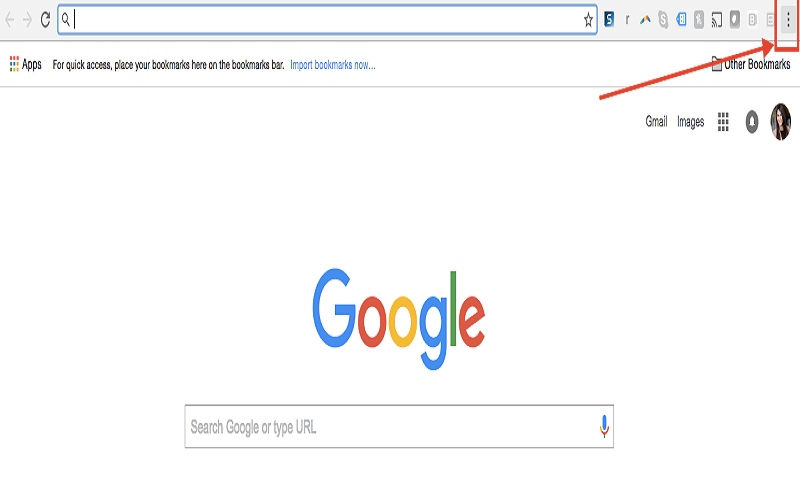This image is a screenshot taken from the Google homepage. Prominently displayed in the center is the recognizable Google logo, with its colorful letters: a blue 'G', a red 'o', a yellow 'o', a blue 'g', a green 'l', and a red 'e'. Below the logo is the search bar, which invites users to "Search Google or type URL." 

At the top of the browser window, in the left-hand corner, are the navigation controls, including the back and forward keys, as well as the refresh button. The URL bar above them is empty, indicating no web address has been entered yet.

In the upper right-hand corner, a red arrow and a red rectangle highlight a small settings button comprised of three vertically aligned black dots. This emphasis suggests that the settings option is essential for the user's attention at this moment.

Overall, the image captures the Google search homepage along with a focus on the browser's settings feature, illustrating the key elements of a typical user’s web browsing experience.